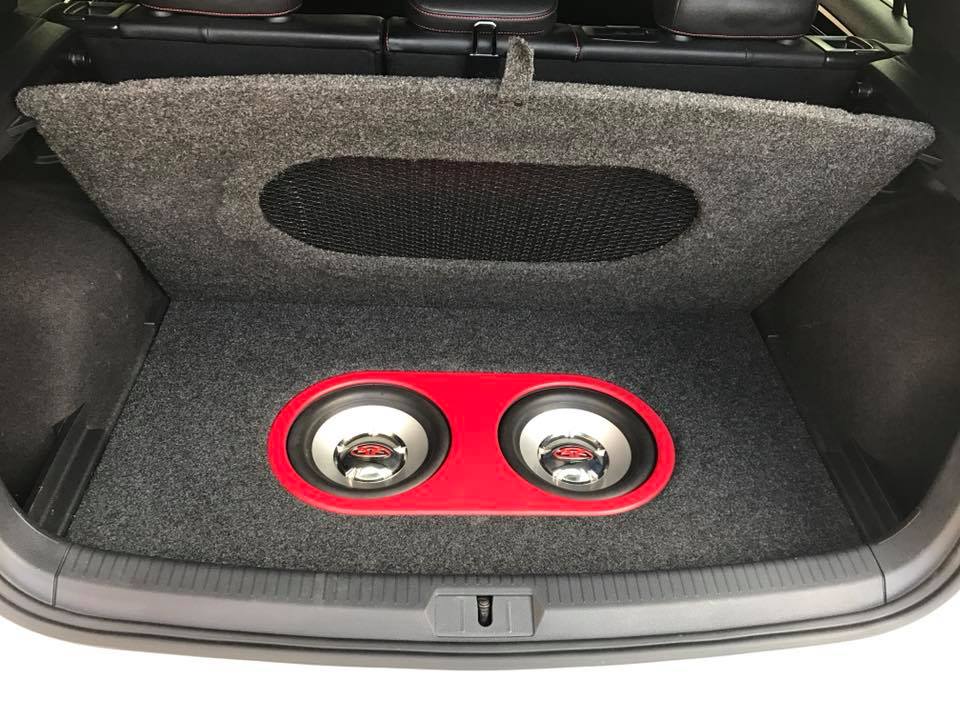This is a detailed image of the trunk area of a seemingly brand new, possibly black hatchback-styled SUV. The trunk is medium-sized with visible gray carpeting. The trunk’s cover, which is also gray, is lifted and features an oval-shaped section of black mesh plastic designed to align perfectly with the subwoofers below. These subwoofers are integrated into the floor of the trunk and are encased in a distinct red border, adding a touch of color to the otherwise monochromatic interior. The leather car seats in the background, glimpsed through the trunk space, have red stitching, further complementing the subwoofers' red trim. The trunk is notably clean, emphasizing the vehicle's newness and the sharpness of the photo captures this detail vividly.